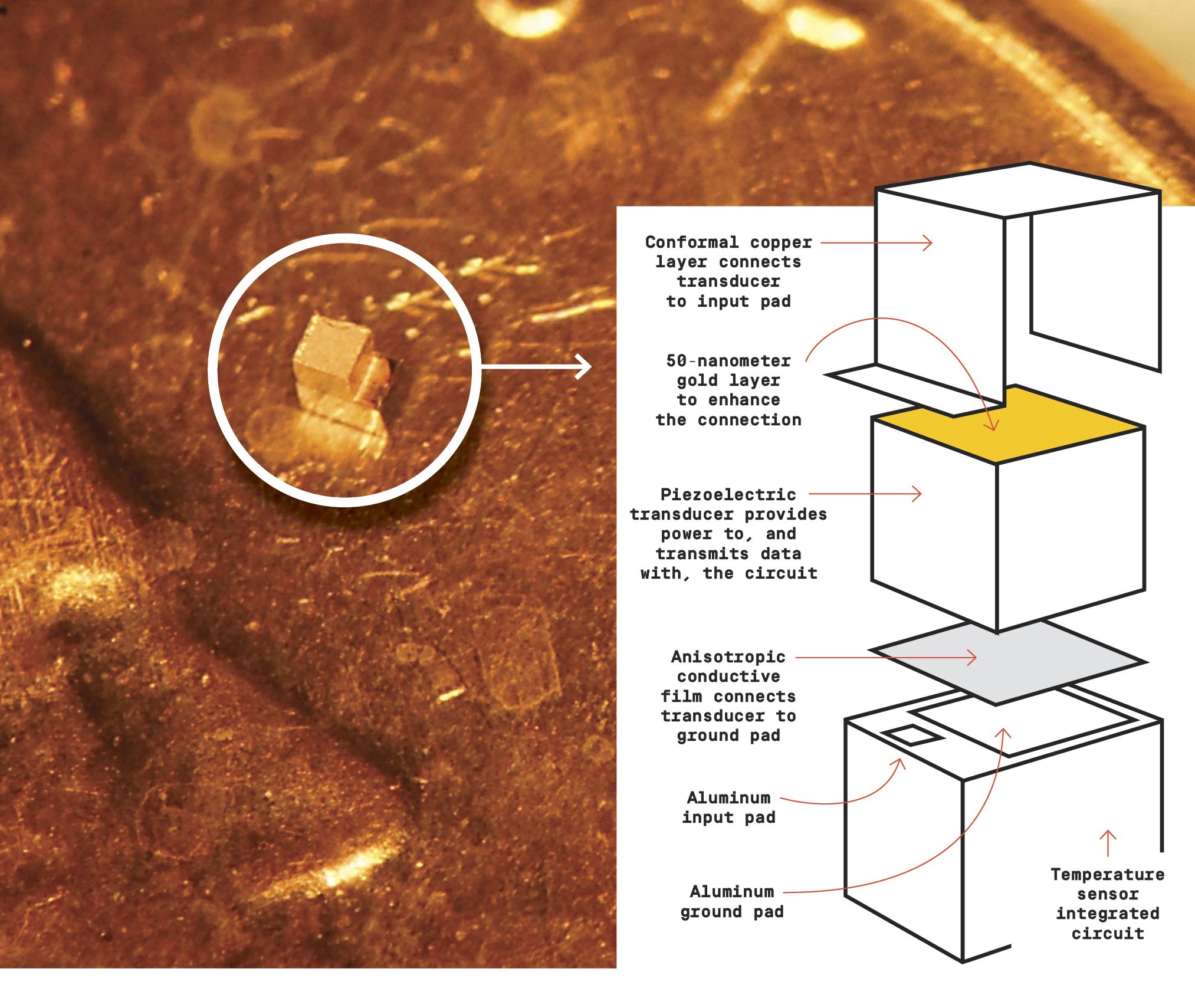The detailed image showcases a golden copper coin displaying the profile of a person's forehead and nose in the lower-left corner. Towards the upper right of the coin's curved edge, two small squares of metal are stacked, forming a rectangular base with a smaller square on top, resembling two steps. This composition is set against a predominantly brown or gold background. An inset diagram occupies the lower right portion of the image. The diagram, outlined with a white circle and connected by an arrow, zooms in on the metal stack and dissects it into multiple labeled layers. These labels detail various features such as conductivity and material composition: the top box is a conformal copper layer connecting a transducer to an input pad; the middle box, with a golden top, is a 50 nanometer gold layer enhancing the connection; supporting layers include a piezoelectric transducer for power and data transmission, an isotropic conductive film, aluminum input and ground pads, and a temperature sensor integrated circuit. The combination of photograph and detailed diagram underscores the technical focus on the layered metal structure and its components.